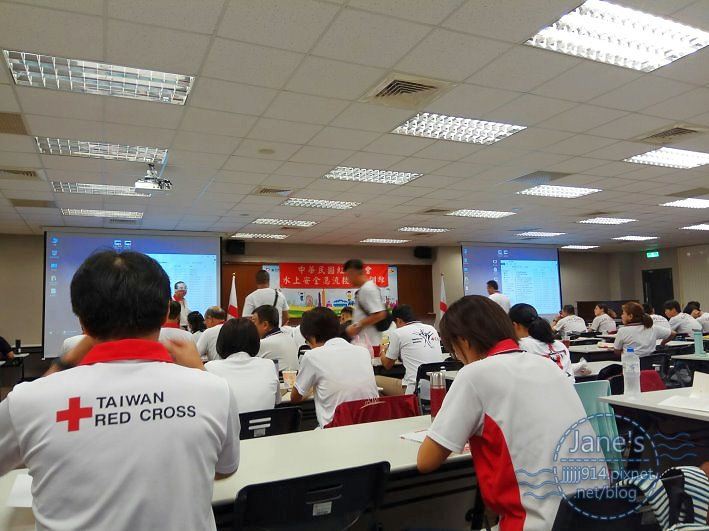The image depicts a classroom filled with numerous students seated at desks, their backs towards the camera. The classroom is equipped with standard AC vents and lighting, and the desks have white tops. The majority of students are wearing white T-shirts that read "Taiwan Red Cross" on the back, accompanied by the Red Cross logo. Both male and female students, who appear to be Asian, are present. Some chairs are black while others are red.

In the bottom left corner, a man with dark black hair wearing a white shirt with a red collar and the words "Taiwan Red Cross" in black text on the back is noticeable. Next to him, at the same table, there is a girl with black hair also wearing a white shirt, which has a black collar and a red section near the ribs.

At the front of the classroom are two large projector screens displaying a white page against a dark blue background, flanked by flags and banners. The banners include one red banner with Chinese writing and others with drawings and paintings. There are also several black boxes, probably speakers, mounted near the ceiling. 

Additionally, some students are standing in the bottom right corner, where a blue circle with the text "janesjjj914.pixpec.net/blog" and decorative swirls is visible. Various colored water bottles are placed on the students' desks, and an exit door is located in the corner of the room. Overall, the setting appears to be a formal educational event or training session, likely related to the Taiwan Red Cross.